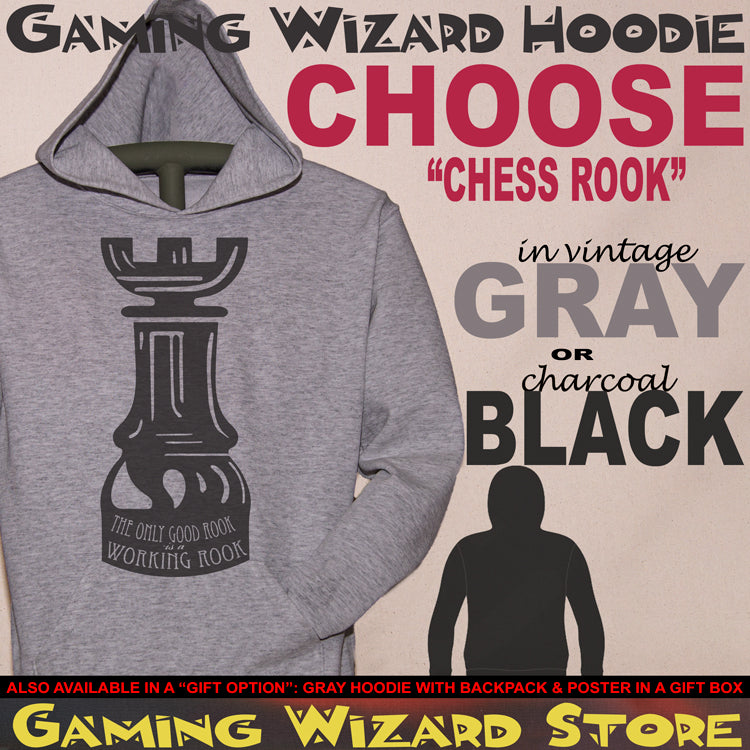This advertisement for the Gaming Wizard store features a prominent light gray hoodie with a dark gray rook design on the front. The rook is accompanied by the slogan "The only good rook is a working rook." The background of the ad is a beige-pinkish hue, with the hoodie positioned on the left side. At the top of the ad, bold black text announces "Gaming Wizard Hoodie," followed by red text "CHOOSE 'CHESS ROOK'." The hoodie is offered in two colors, with "Vintage Gray" and "Charcoal Black" highlighted in corresponding colored fonts. Below the text descriptions is an image of the hoodie in each color option. At the bottom of the ad, red text states, "Also Available in a Gift Option: gray hoodie with backpack and poster in a gift box." The bottom of the ad features the store name, "Gaming Wizard Store," in yellow capital letters. This detailed and visually engaging ad is designed to attract online shoppers looking for stylish and thematic chess apparel.